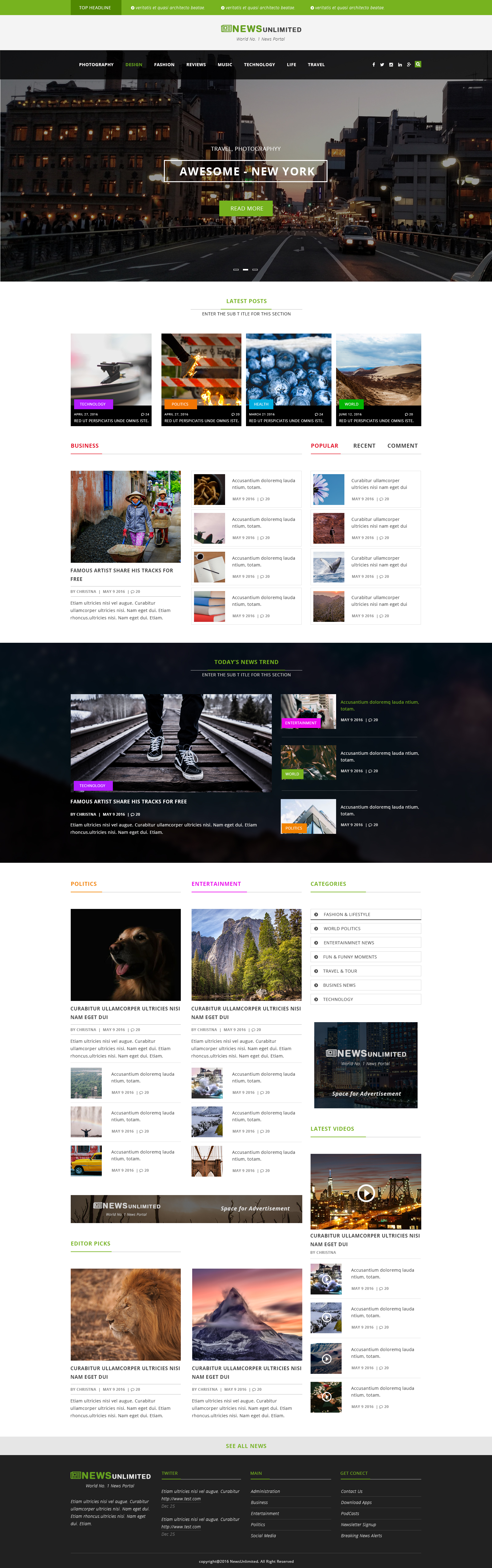This image is a screenshot from an unidentified website. At the very top, there's a very thin strip of lime green, followed by a white banner with illegible text. Directly below the banner is the header graphic, featuring a city street scene. In bold, white capital letters, the text "AWESOME NEW YORK" is prominently displayed, suggesting the content relates to New York City, potentially downtown or Soho.

Beneath the header graphic is a section with a white background containing various small photos, likely landscapes. Below this array, there is another set of even smaller photos arranged in a column, each accompanied by writing on the right, though the text is too small to decipher.

In the center of the webpage is a striking photo: a close-up of railroad tracks with someone's feet and lower pant legs visible. The individual is wearing black sneakers and black pants. The area surrounding this central photo features a black background.

At the bottom of the screenshot, the background returns to white, displaying multiple series of smaller photos accompanied by text summaries, though again, the writing remains too small to read.